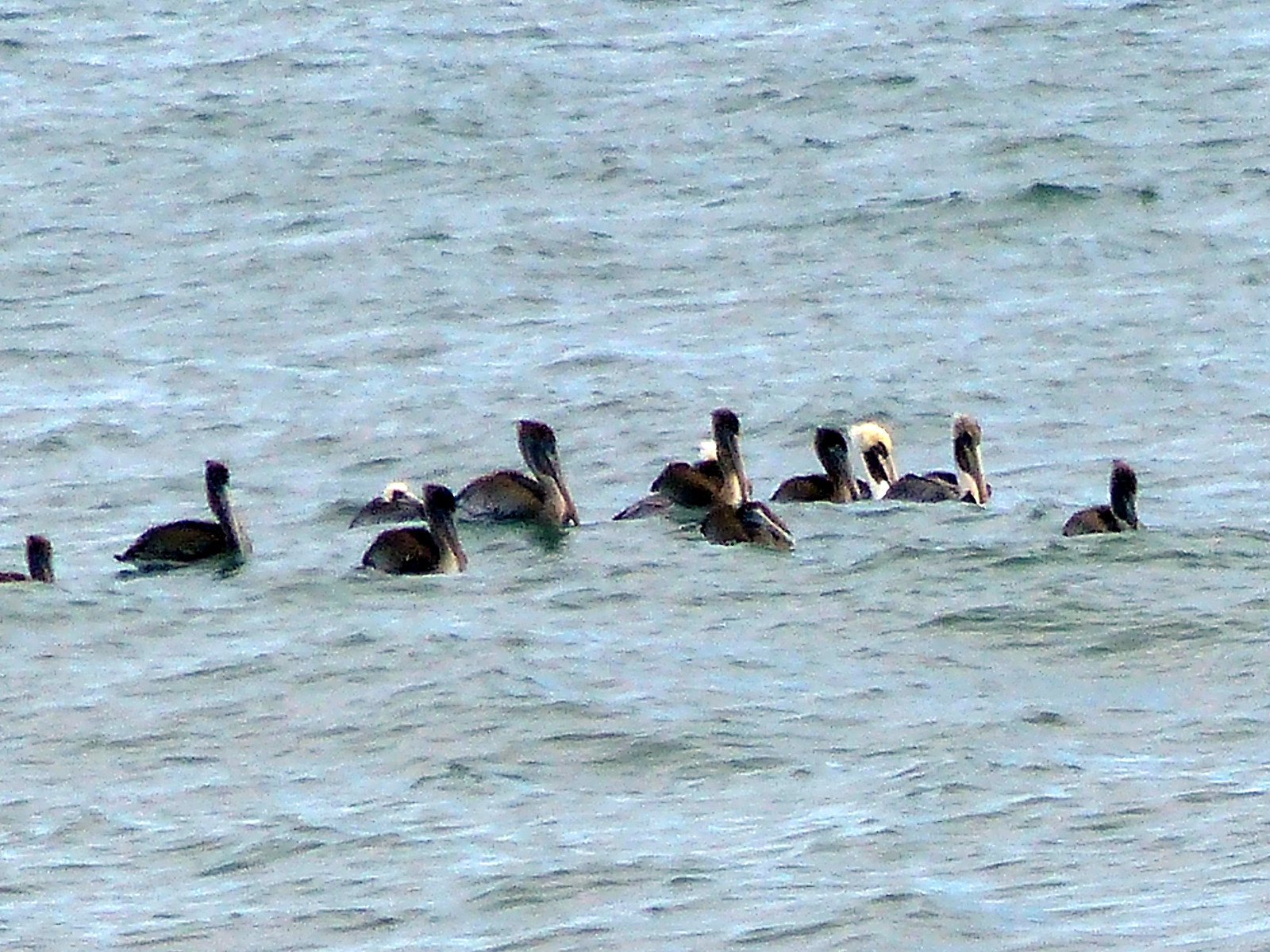The image is an outdoor scene depicting a choppy, dark blue lake filled with pelicans and seagulls. There are 12 pelicans clearly visible, mostly dark in color, with three distinct ones having white heads framed by black around their faces. Additionally, there are 11 seagulls amidst the pelicans, all moving from the left to the right side of the frame. The seagulls exhibit varied appearances: one has a black body with its head straight up in the air, another has a white head, and others show a mix of gray and black feathers. Notably, a larger seagull with a greenish head and gray body stands out, accompanied by a smaller, similar-looking seagull. Some seagulls appear more submerged, blending into the waves, while others have their beaks down to their chests, contributing to the dynamic and bustling atmosphere as they all navigate the lively waters together.